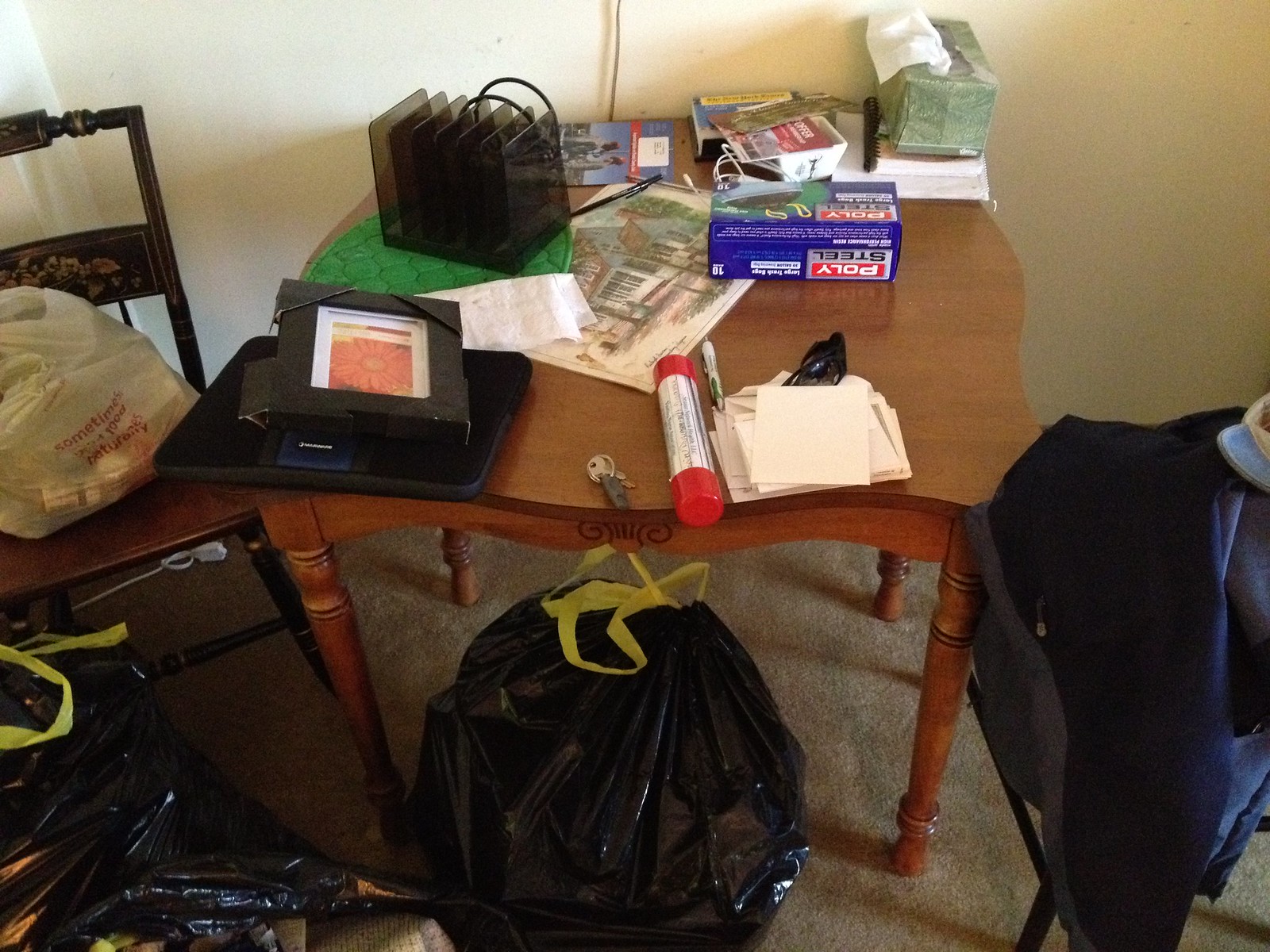The image depicts a cluttered scene within what appears to be a small, untidy apartment. Dominating the foreground is a brown wooden table, heavily laden with various items including keys, paper, a pen, Poly Steel packaging, Kleenex, and a picture frame. To the left of the table stands a chair, which currently holds a grocery bag filled with unspecified items. Underneath the table, slightly towards the front, is a full trash bag, and another full trash bag is positioned near the chair to the left.

The table rests atop a light tan carpet, which further extends to the surrounding area. On the right side of the table, the legs of another chair are visible, the seat itself obscured by a pile of dark navy blue and gray clothing. The overall atmosphere conveyed by the image is one of disorganization and neglect, as indicated by the scattered belongings and the overflowing trash bags.